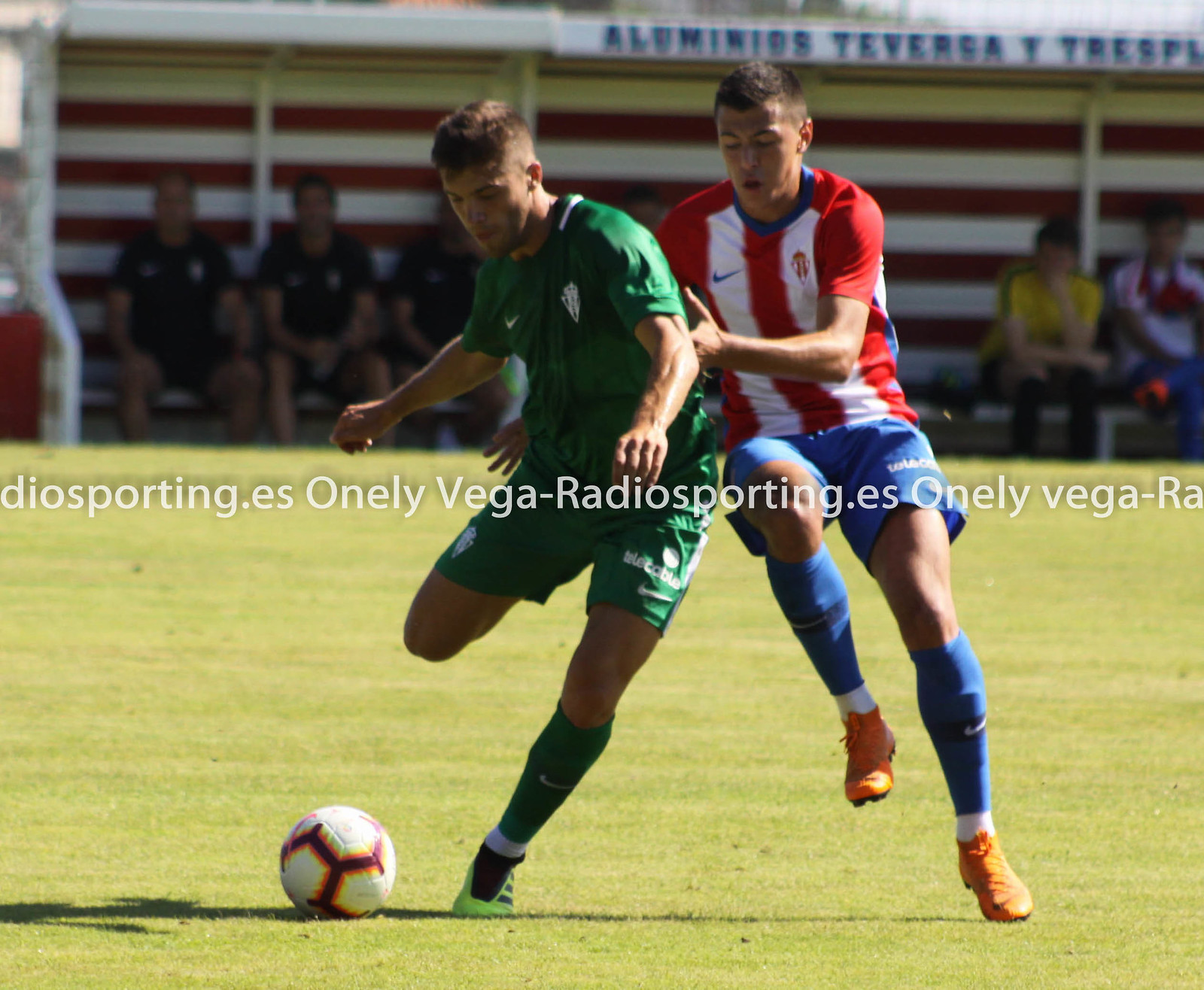This action-packed photograph captures a dynamic moment in a soccer match between two players from opposing teams on a lush green grass pitch. The player on the left, who is dressed in a medium green uniform with matching socks and light green cleats, has planted his left foot firmly on the ground and is leaning backwards, poised to kick the ball with his right foot. Meanwhile, his opponent, wearing a red and white vertical striped jersey, blue shorts, blue socks, and orange cleats, is closing in on him. This player is mid-stride, with his right foot off the ground and his left arm bent at a 90-degree angle, seemingly about to make a defensive play by intersecting or blocking the kick. Both players are intensely focused on the ball, which lies on the ground between them.

In the distant background, a group of individuals, possibly other players or spectators, are seated under a dugout with an awning. The dugout has a sign in blue text that reads "Alumnios Tavrega e Trisbo" and appears to be sheltering the onlookers from the sunlight visibly reflecting off the grass. The photograph also features a watermark text, "onlyvegaradiosporting.es," repeated across the image. This detailed and vivid imagery encapsulates the competitive spirit of the game.